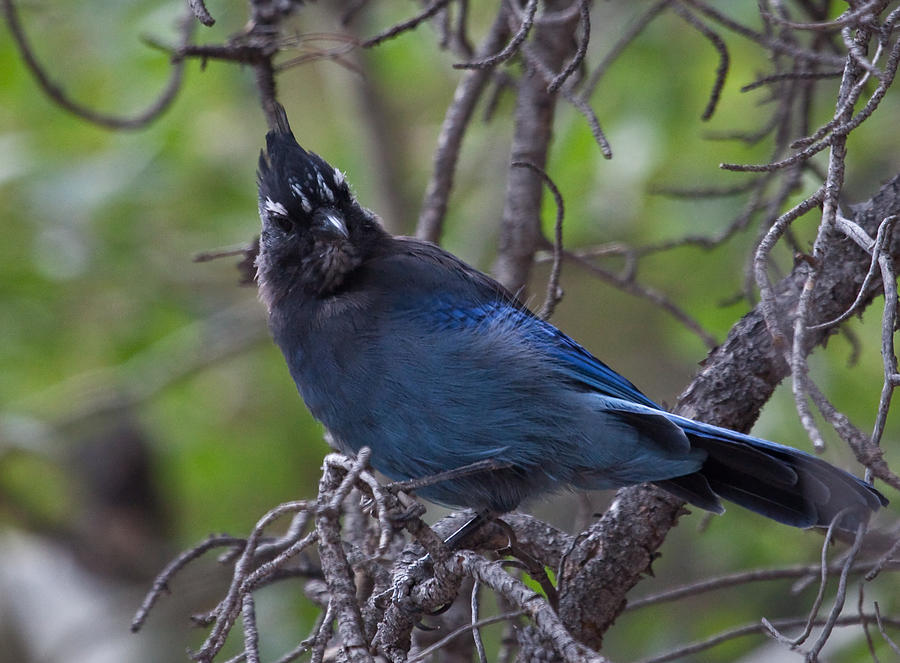This photograph captures a detailed, close-up shot of a blue bird, possibly a blue jay, perched on a gnarled, dark tree branch amidst a lush, woodland setting. The bird's plumage features a striking blend of black and various shades of blue, ranging from a shimmering light blue on its wings and tail to a very dark navy blue on its body. Its head, accentuated by fluffy feathers, is black with four clusters of tiny white markings, especially around and above its black eyes, which add a touch of contrast. The bird's head is turned almost 180 degrees, gazing directly at the camera, showcasing its small, curved beak that hints at a diet of nuts or fruits.

The background is artfully blurred, employing a bokeh effect that highlights the bird and the rugged texture of the branch while subtly indicating a green, leafy environment. The tree branch on which the bird is perched has several offshoots, creating a complex and natural frame around the bird. The scene suggests an autumn or winter season, as the tree is devoid of leaves. The overall composition draws the viewer's eye directly to the bird, emphasizing its vibrant colors and intricate details against a soothing, diffused backdrop.